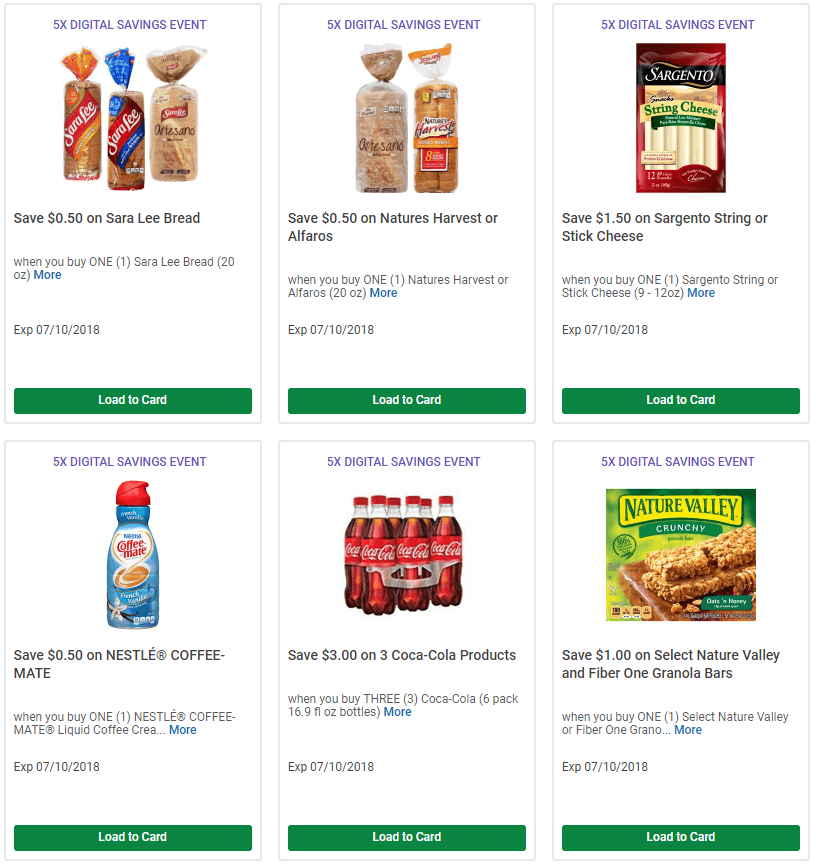The image depicts an online store featuring a variety of food products on promotion. The store's name isn't specified, but several enticing deals on food items are prominently displayed. 

1. **Sara Lee Bread**: A promotion highlighting a discount, where you can save 50 cents on Sara Lee bread when you buy one or more. The banner above the image reads "Five Times Digital Savings Event" in purple.

2. **Nature's Harvest or Alfaro's Bread**: Another deal showcases a 50-cent savings on Nature's Harvest or Alfaro's bread when you purchase one. Again, the banner above reads, "Five Times Digital Savings Event" in purple.

3. **Sargento String or Stick Cheese**: This deal offers a $1.50 savings on Sargento string or stick cheese. The same purple banner, "Five Times Digital Savings Event," is displayed above the image.

4. **Nestle Coffee Mate**: At the bottom, there's a promotion for a 50-cent discount on Nestle Coffee Mate. The familiar purple "Five Times Digital Savings Event" banner is visible above.

5. **Coca-Cola Products**: A significant discount where you can save $3 when you purchase three Coca-Cola products. The purple banner indicating "Five Times Digital Savings Event" appears above.

6. **Nature Valley and Fiber One Granola Bars**: The final deal offers a $1 discount on select Nature Valley and Fiber One granola bars. The same purple "Five Times Digital Savings Event" banner is present above the product image.

Each deal can be conveniently loaded to your card, indicated by green bars beneath each promotion, allowing for easy digital savings activation.